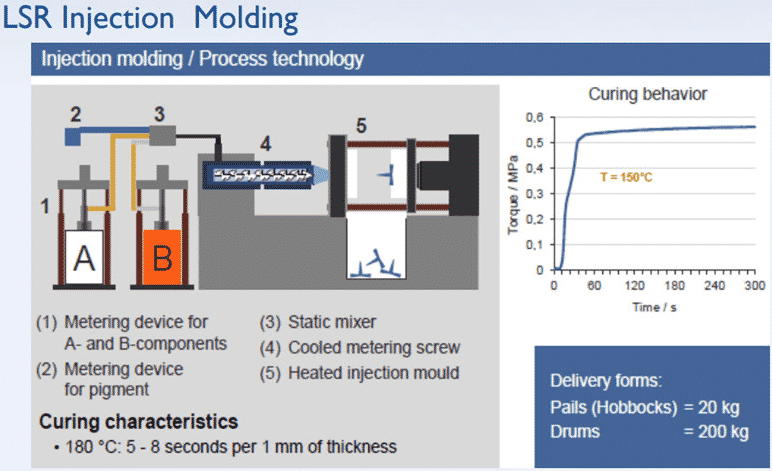This detailed diagram, likely from a technical book, explains the LSR (Liquid Silicone Rubber) Injection Molding process. The top left of the image prominently titles it "LSR Injection Molding," followed by a subheading "Injection Molding / Process Technology" with a blue background. Below this, the diagram outlines the injection molding process, featuring components colored and numbered for clarity.

Component A (white) and Component B (orange) are both directed into a "Metering Device for A and B components" (1). They are then mixed with pigment in the "Metering Device for Pigment" (2), followed by passage through the "Static Mixer" (3). The blend moves into the "Cooled Metering Screw" (4) before finally reaching the "Heated Injection Mold" (5), which outputs the molded product.

Additionally, curing characteristics are specified: 180 degrees Celsius, with a curing time of 5 to 8 seconds per 1 mm thickness. To the right of the diagram, a graph labeled "Curing Behavior" maps the relationship between Torque/MPA and Time in seconds (0 to 300), with the y-axis ranging from 0 to 0.6 and a highlighted line indicating T = 150 degrees Celsius.

At the bottom right, a blue box labeled "Delivery Forms" specifies the packaging options: Pails (Hobbux) containing 20 kg and Drums containing 200 kg. The detailed visual aids, including colors, numbers, graphs, text descriptions, and equations, suggest that specialized training is required to fully understand the technical aspects presented.